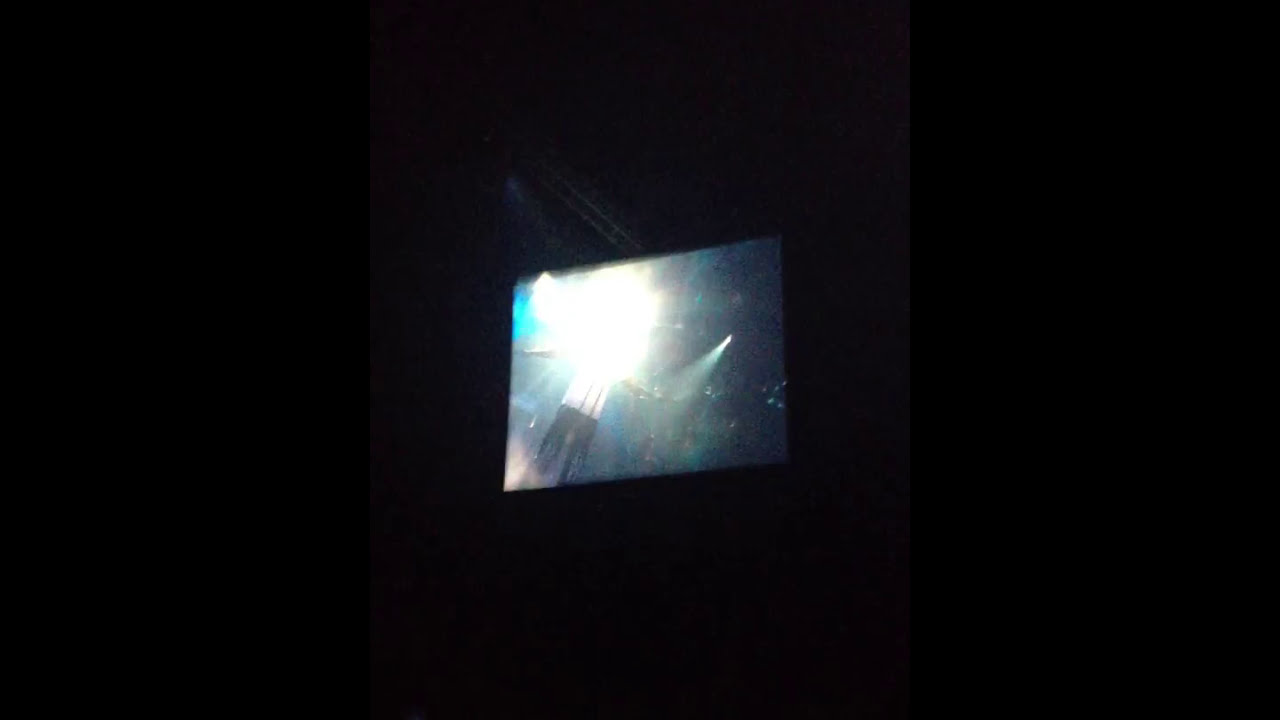A photograph captures a square screen with a celestial backdrop of stars set against the black night sky, all framed within a larger expanse of pure black that extends to the left, right, top, and bottom. The screen is positioned centrally, both horizontally and vertically. An intense flash of light, likely from the camera, obscures the face of a person standing with their arms extended within the screen. The image on the screen seems to depict either a movie or TV show still, where the colors range from gray to bluish hues. The background wall that the screen is mounted on remains indiscernible due to the overwhelmingly dark surroundings. The screen itself appears at a slight diagonal angle, with the lower part touching the left edge and the upper part angled slightly upward to the right.